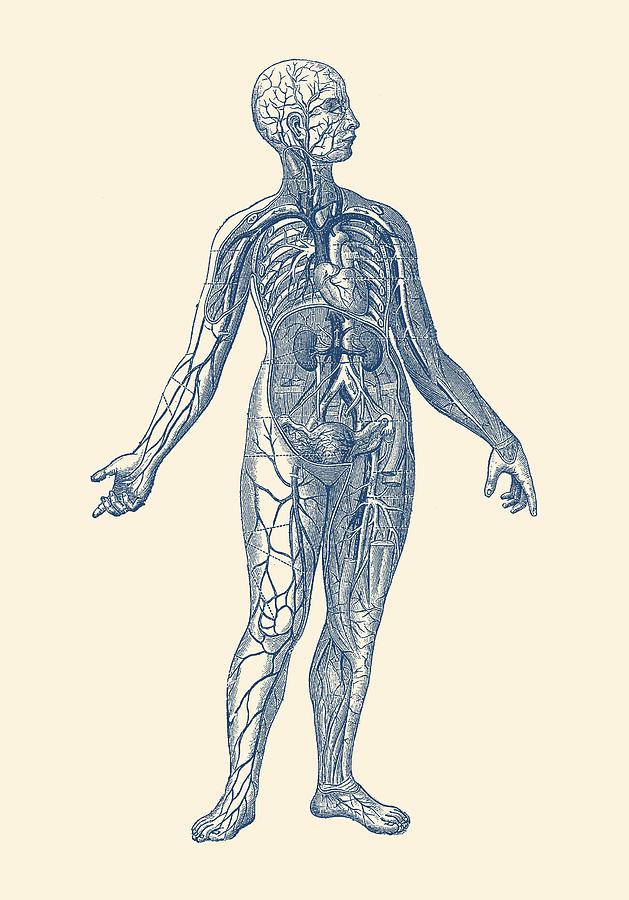This detailed anatomical illustration, likely from an anatomy or medical textbook, presents an in-depth view of the human circulatory system. Set against a tan background, the finely detailed diagram showcases a human figure facing slightly to the right with arms extended outwards, emphasizing the extensive network of blood vessels throughout the body. The heart, centrally located in the torso, is prominently displayed, accompanied by detailed illustrations of the kidneys, major veins, and arteries. The diagram also reveals other critical anatomical features such as the lungs, skeletal structure, and muscles, with certain sections cut away to provide a clear view of the underlying veins and arteries. Veins ascend to the brain and descend through the legs and arms, prominently displayed to trace the path of blood flow. Notably, the illustration highlights major veins in the legs and arms, providing a comprehensive understanding of blood distribution in the human body.